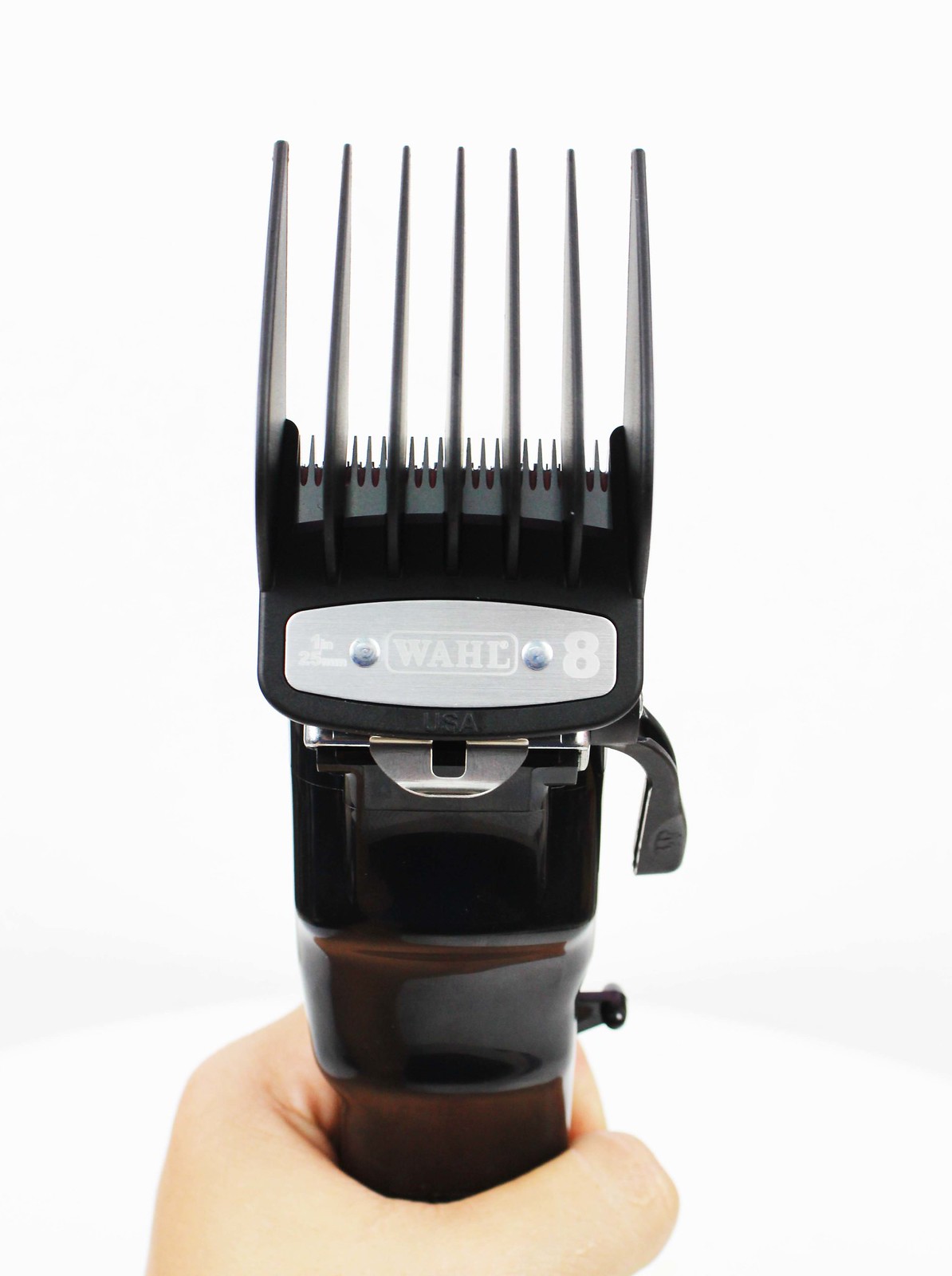In this detailed photograph, a pale, white hand firmly grips the base of a pair of Wahl electric hair clippers, which are characterized by a deep, dark plastic resembling wood. The hand, positioned at the lower part of the clippers, wraps around the handle with the thumb and knuckle visibly prominent. The clippers themselves are primarily black with a notable silver plate affixed in the middle. This plate bears the clearly readable "Wahl" brand logo encased in a box, accompanied by a number eight, indicating the guard attached to the clippers. The number eight guard features long, thin tines suitable for shaping hair or trimming beards to a specific length. Additionally, the clippers are equipped with a small black handle on the side for adjusting the cutting depth and fine-tuning the length. The background of the image is a light gray, contrasting slightly with the display screen, and emphasizing the form of the clippers.